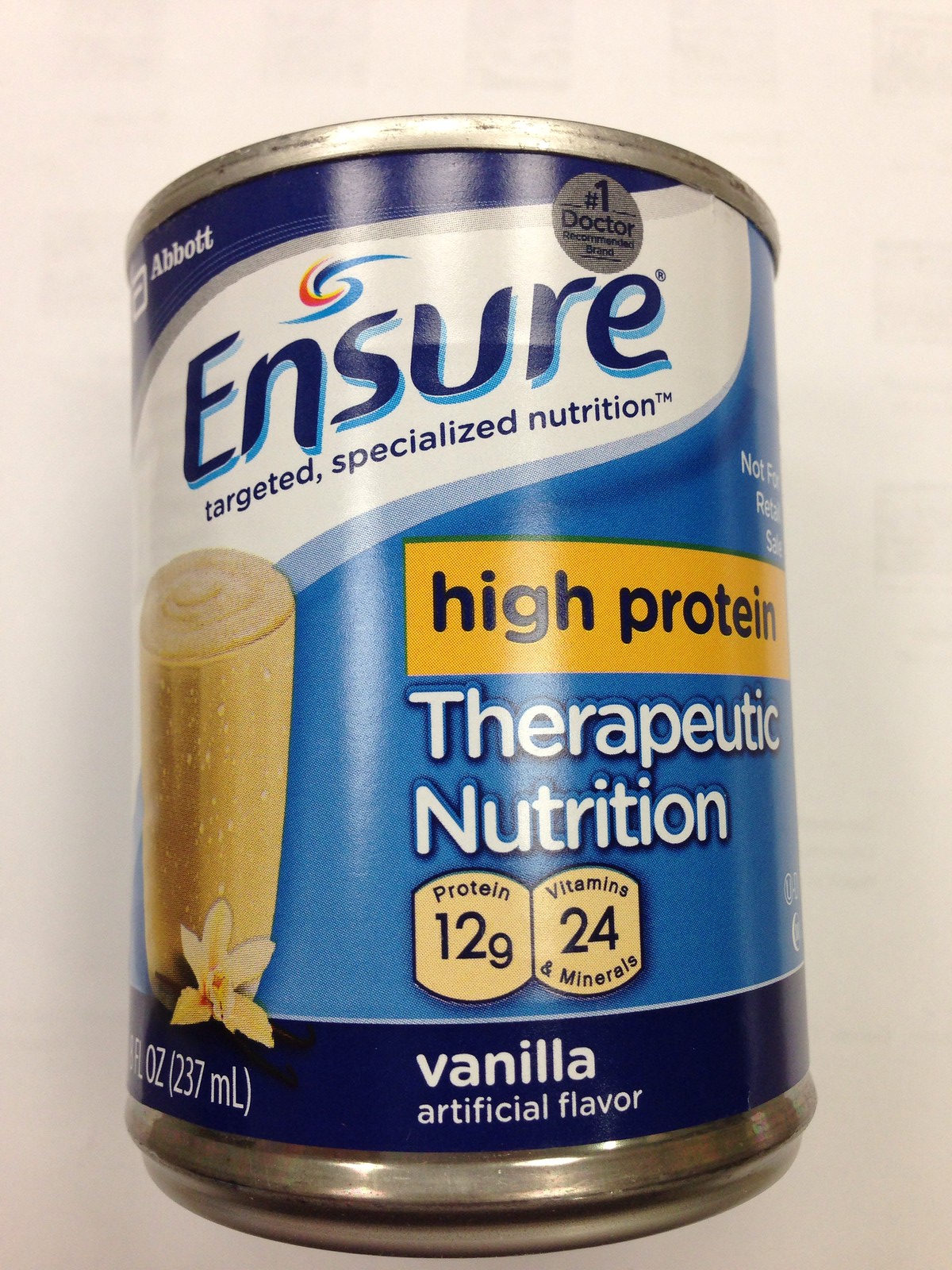The image depicts a can of Vanilla Ensure, which is a high-protein nutritional drink. The can features a multi-tone blue label with white accents and prominently displays the Ensure logo across the front. Below the logo, there's a representation of a light beige to off-white drink in a cup, accompanied by a vanilla flower, highlighting the vanilla artificial flavor at the bottom of the label. The label also includes key nutritional information, such as "High Protein Therapeutic Nutrition" with 12 grams of protein and 24 vitamins and minerals. Additional text indicates that this product is the "#1 Doctor Recommended Brand," with this endorsement appearing in a silver and blue badge near the top. The can also features a yellow banner that reads "High Protein" and specifies that it contains 237 milliliters (8 ounces) of liquid. There's a note near the top stating "Not for Retail Sale," implying it is part of a larger package. The entire setting is placed against a plain white background.